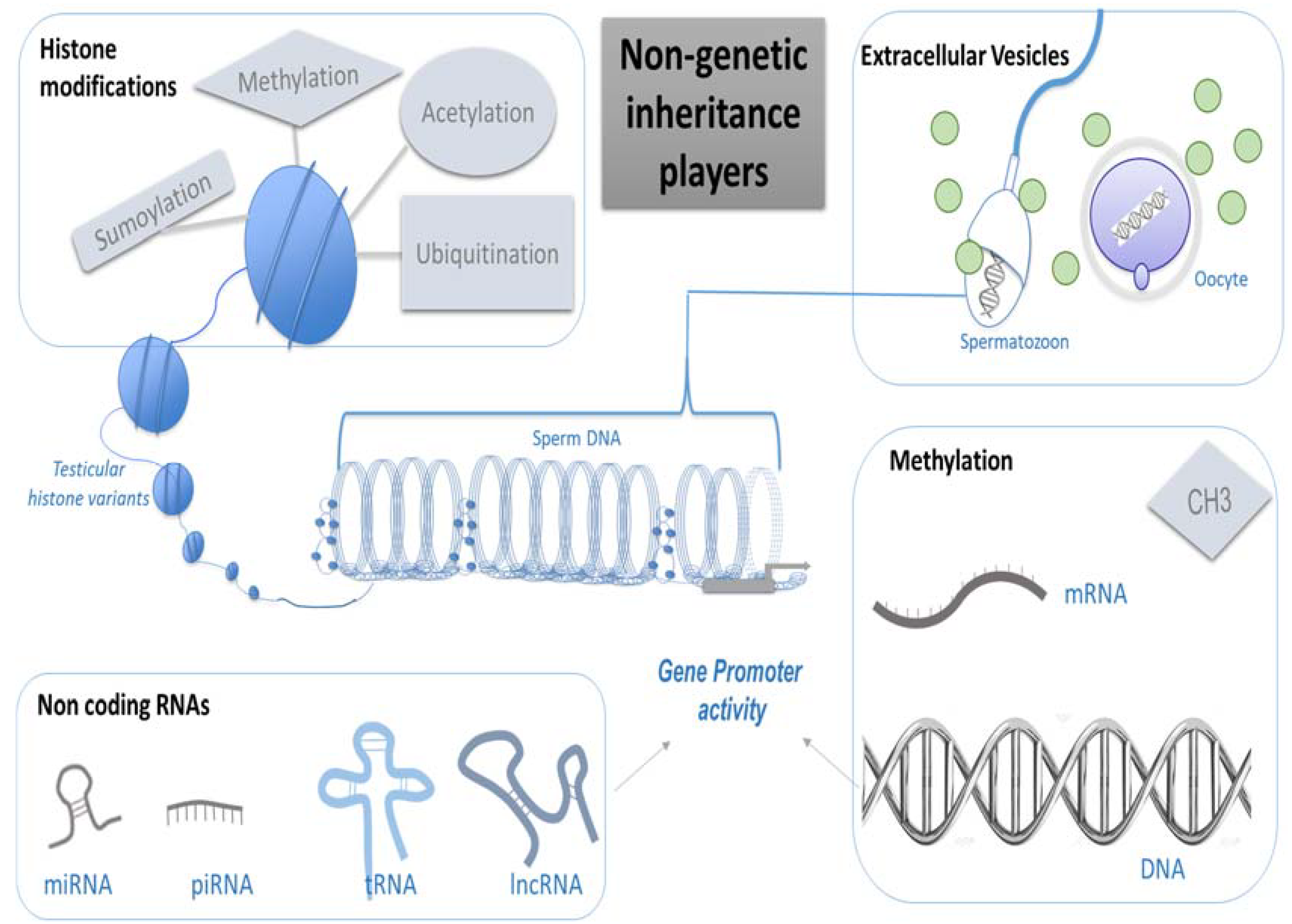The image is a detailed scientific diagram highlighting key components involved in non-genetic inheritance. At the top center, a gray box titled "Non-Genetic Inheritance Players" sets the theme. The diagram is divided into four sections. The upper left section, marked "Histone Modifications," features blue ovals labeled with histone-related terms and pathways leading to shapes tagged with "Testicular Histone Variants." The upper right section, labeled "Extracellular Vesicles," includes green circles representing oocytes and sperm. The bottom left area is dedicated to "Non-Coding RNAs," illustrating various RNA structures with labels and connections to "Gene Promoter Activity." The lower right section, titled "Methylation," portrays DNA and mRNA imagery along with a box labeled "CH3" to indicate methylation. Central elements like "Sperm DNA" connect these sections, emphasizing interaction among the various non-genetic inheritance mechanisms. The diagram is color-coded with white, blue, gray, purple, and green, providing a clear, visual account of the complex biological concepts.